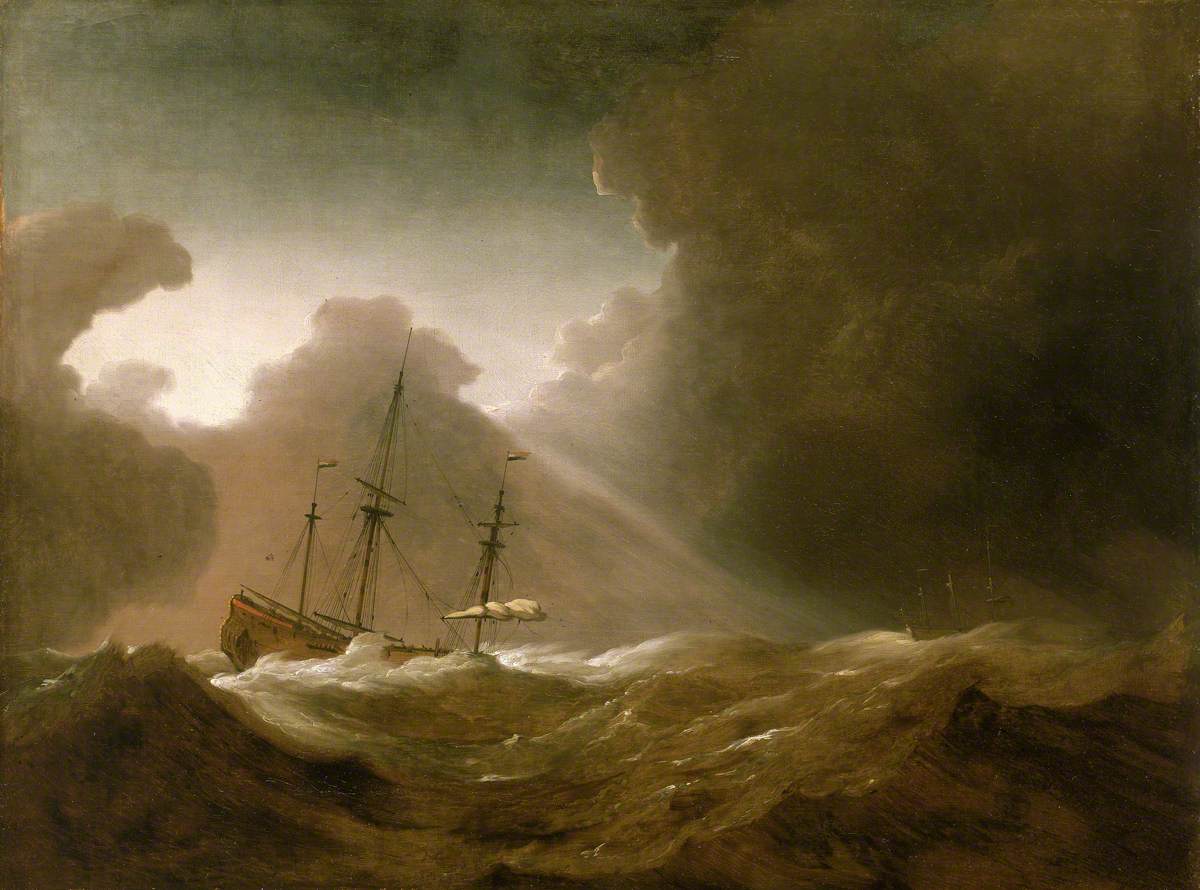The artwork is a highly detailed and dramatic seascape illustration, capturing a turbulent scene where a pirate ship battles against a raging storm. The central focus of the image is the beleaguered ship, immersed in crashing waves that obscure much of its hull, leaving only the mast and a few tattered sails visible. The sea is tumultuous, with large waves cresting into whitecaps, emphasizing the ferocity of the storm. In the foreground, turbulent waves with frothy tops add to the sense of chaos. 

The background features a foreboding, stormy sky dominated by thick, swirling clouds that mirror the movement of the sea below. A massive black cloud looms ominously in the upper right corner, while a small sliver of light attempts to pierce through the clouds on the left side, adding a stark contrast to the otherwise dark and moody palette. The overall color scheme is muted and dark, enhancing the dramatic and perilous atmosphere as the ship struggles to stay afloat in the relentless storm.